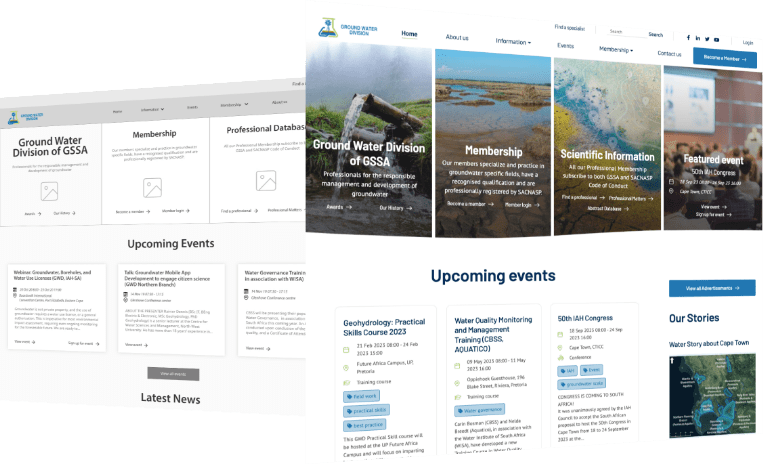The image displays two different webpages from the same website, each centered around water resources and hydrology. 

### Foreground Webpage:
- **Title**: Groundwater Division of GSSA
- **Visuals**: This page prominently features four images, each depicting a waterway. The images provide a dynamic visual representation with flowing water and are potentially related to various topics under the Groundwater Division.
  - The first image shows the actual water flow within a waterway.
  - The second image highlights a membership section, again illustrated by a waterway.
  - The third image offers a scientific perspective from an aerial view of a waterway.
  - The fourth image is designated for a featured event.
- **Navigation and Layout**: 
  - Across the top, there are six navigation tabs labeled numerically from 1 to 6, alongside the website name and logo, although the latter is not clearly readable.
  - The body of the webpage features sections for upcoming events which are outlined with checkboxes, texts, and interactive buttons.
  - Upcoming events include:
    - **Geohydrology Practical Skills Course 2023**: A designated box with checkboxes and buttons for further actions.
    - **Water Quality Monitoring and Management Training by CBSS Aquatico**: Descriptive text accompanied by checkboxes and a button.
    - **50th IAH Congress**: Contains three checkboxes, four interactive buttons, and relevant text information.
- **Right Side Content**: A section titled "Our Stories".

### Background Webpage:
- **Comparison**: Provides a skeletal structure of the same webpage layout seen in the foreground but without the visual images and detailed text, illustrating the development process from the barebones template to the fully constructed webpage.

In summary, the image reflectively portrays two states of website interface—one a detailed, image-rich final product, and the other, a preliminary, plain layout, emphasizing the stages of webpage development.